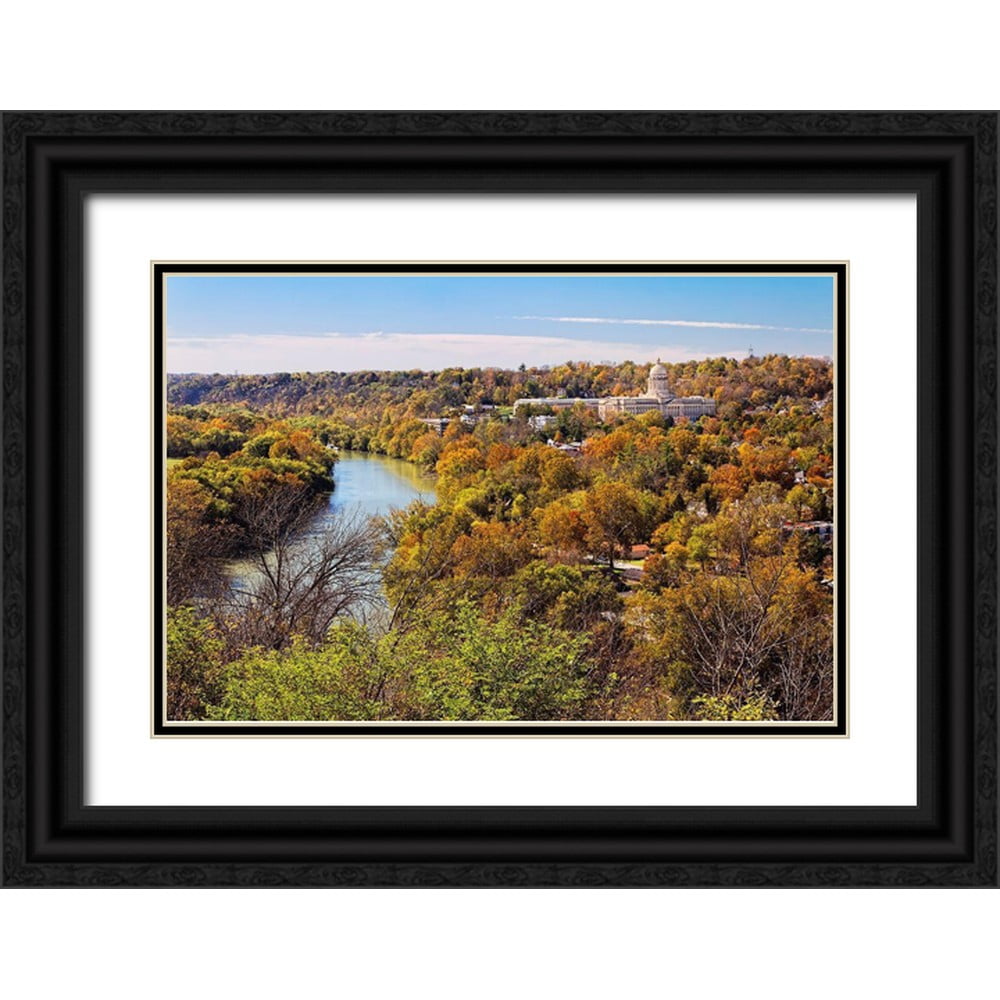This framed photograph, elegantly encased in a black frame with a white border and black matting, captures a vibrant autumn landscape. The central image showcases a serene fall scene where trees display a kaleidoscope of colors: deep greens, fiery reds, gleaming golds, and sunlit oranges. The foliage is in varying stages of fall, with some trees already bare. Dominating the left side of the picture, a reflective body of water, possibly a river or creek, mirrors the bright blue sky above, which is adorned with a few wispy white clouds. Dotted amongst the trees, slight hints of a neighborhood emerge with tiny white houses, contributing to the pastoral charm. In the backdrop, a distinguished white building with a dome—possibly resembling a capitol or courthouse—stands out, woven seamlessly amongst the trees, completing this picturesque and tranquil autumnal scene.